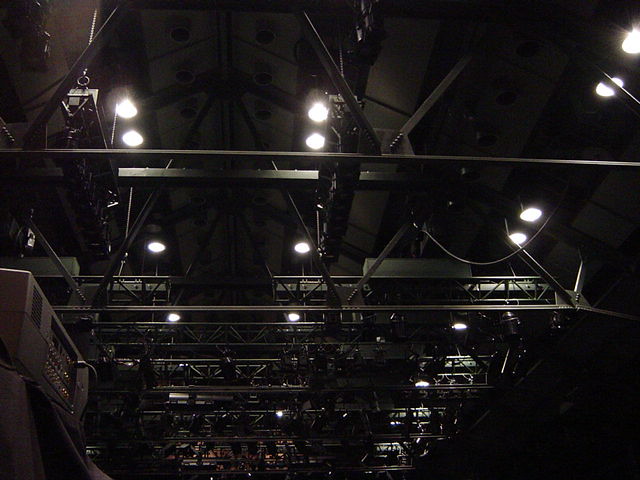This image is a highly detailed photograph taken inside a dark, indoor space, such as an industrial plant, warehouse, or the back of a theater. The photograph, which may be in color or black and white, emphasizes a complex arrangement of professional lighting and structural elements. 

The ceiling is exceptionally high and features a network of dark-colored support beams and steel apparatus, forming a grid of triangular tubing, bridges, and catwalks. Suspended from this intricate framework are numerous round white spotlights arranged in long rows, illuminating the floor below with bright, focused beams. 

On the left side of the image, there is a structure resembling a control center or a flat surface covered in black cloth, accompanied by a piece of sound equipment with a visible cable plugged in. The image captures the ceiling extending beyond the frame, showcasing the expansive and vaulted architecture of the room. Despite the floodlights, the photograph remains dark, highlighting the stark contrast between the lit areas and the shadowed, industrial ambiance.